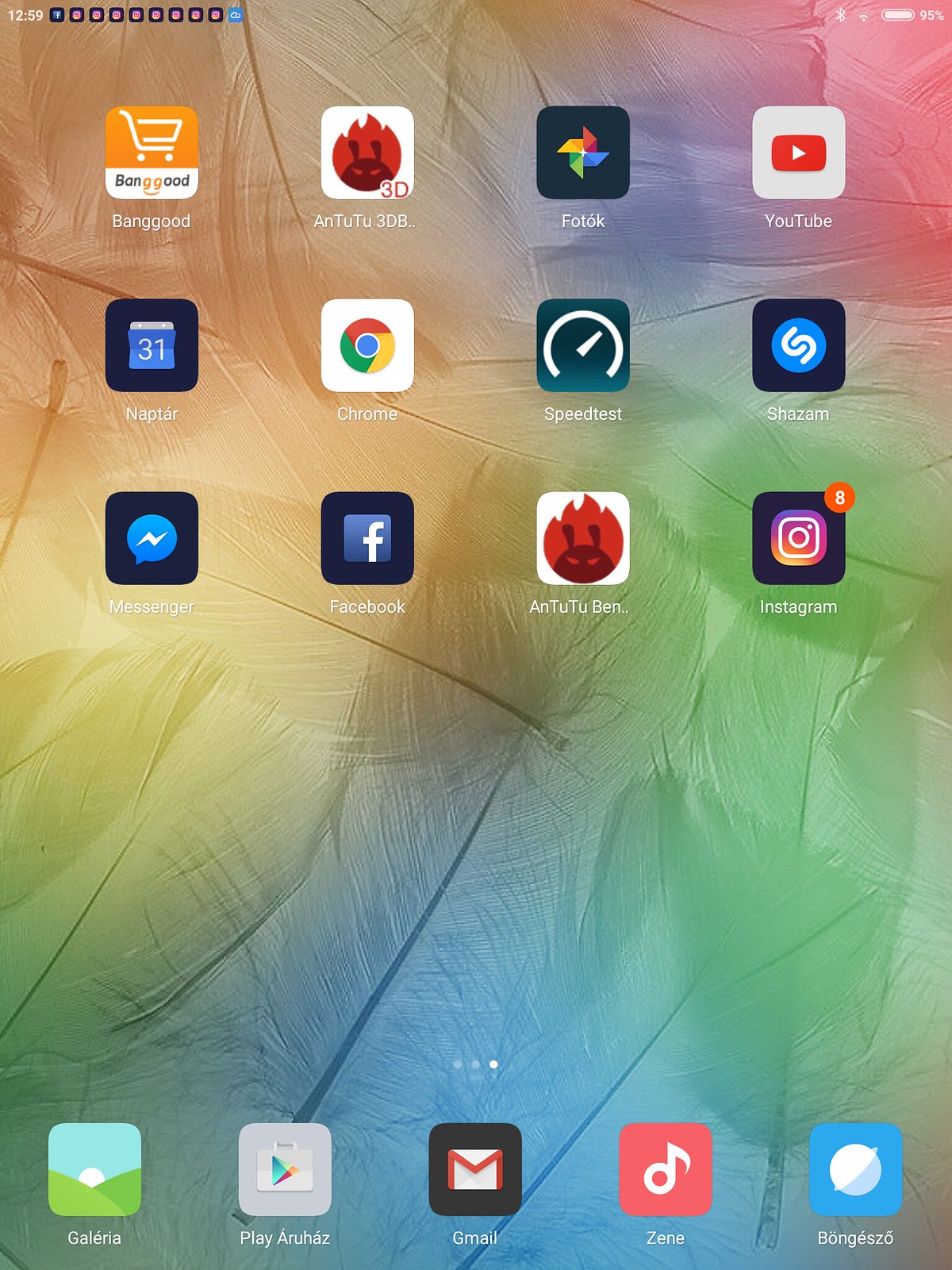Here is a detailed and cleaned-up caption for the given image:

"This screenshot captures the home screen of an Android tablet. In the top left corner, the time is displayed as 12:59, accompanied by various status icons indicating a 50% Wi-Fi signal strength, Bluetooth being enabled, and a battery level at 95%. 

The notification bar shows multiple app notifications, including Facebook, Instagram (repeated eight times), and an icon resembling a blue cloud.

The main screen is populated with various app icons arranged in a grid format. The visible apps include Banggood, Antutu 3DB (possibly a benchmark app), Photoc, YouTube, Naptar (displaying a calendar icon), Chrome, Speedtest, Shazam, Messenger, Facebook, Antutu BEN, and Instagram with eight new notifications. 

At the bottom row, there are additional apps: Galleria, Play Ahra's, Gmail, Zine (spelled Z-E-N-E), and an unknown app icon featuring a blue background with a white circular planet symbol labeled B-O with umlauts, N-G-E-S-Z-E-N-E, B-O."